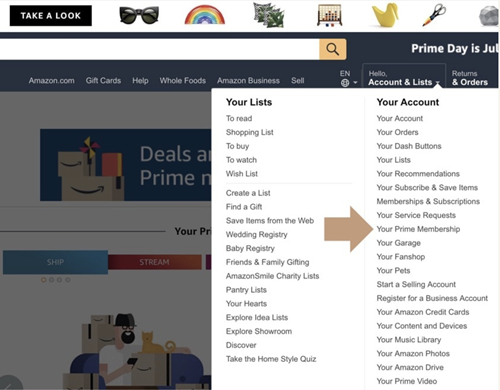The image depicts a partially captured screenshot of an Amazon webpage, specifically focusing on the "Accounts & Lists" section. At the top, there's a prominently visible dark blue banner featuring various Amazon services: "Amazon Gift Cards", "Help", "Whole Foods", "Amazon Business", and "Sell". To the right of these services, the banner reads "Hello" and directly beneath it, "Accounts & Lists" is highlighted in bold white text, indicating it is the current selection. Farther right, "Returns & Orders" is also presented in bold white text, contrasting with the standard white text of the rest of the banner content.

Below the "Accounts & Lists" heading, the section is populated with an array of options under "Your Account," with each option serving a different purpose. A prominent beige arrow directs attention specifically to "Your Prime Membership." The list of options under "Your Account" includes:

1. Your Account
2. Your Orders
3. Your Dash Buttons
4. Your Lists
5. Your Recommendations
6. Your Subscribe and Save Items
7. Memberships and Subscriptions
8. Your Service Requests
9. Your Prime Membership
10. Your Garage
11. Your Fan Shop
12. Your Pets
13. Start a Selling Account
14. Register for a Business Account
15. Your Amazon Credit Cards
16. Your Content and Devices
17. Your Music Library
18. Your Amazon Photos
19. Your Amazon Drive
20. Your Prime Video

To the left, there is a section titled "Your Lists" which includes:

1. To Read
2. Shopping Lists
3. To Buy
4. To Watch
5. Wish Lists
6. Create a List
7. Find a Gift
8. Save Items from the Web
9. Wedding Registry
10. Baby Registry
11. Friends and Family Gifting
12. Amazon Smile Charity Lists
13. Pantry Lists
14. Your Hearts
15. Explore Idea Lists
16. Explore Showroom
17. Discover
18. Take the Home Style Quiz

The screenshot appears to be cropped, not displaying the full breadth of the webpage, which narrows the focus to these detailed account options and list management features.